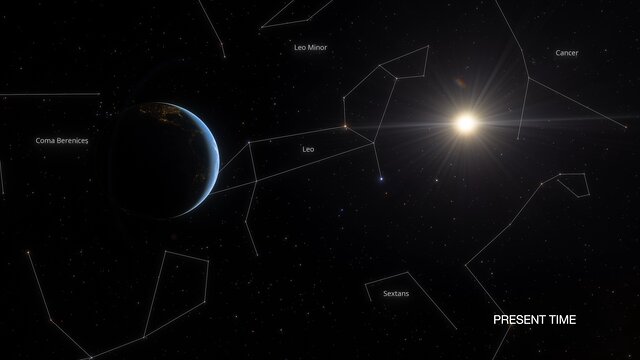The image depicts a detailed star map set against a dark background, representing various constellations in the sky within the solar system. Prominently, it labels and illustrates the constellations of Coma Berenices on the left, Leo in the center, Leo Minor, Cancer in the upper right, and Sextans. The map includes a sliver of the moon on the left side and the sun on the upper right, emitting distant rays. A blue planet, possibly Earth, is visible in the foreground with light reflecting off its surface from the distant, shiny sun. The constellations are connected by thin, pale, white lines between the bright stars, with the bottom right labeled as "present time."